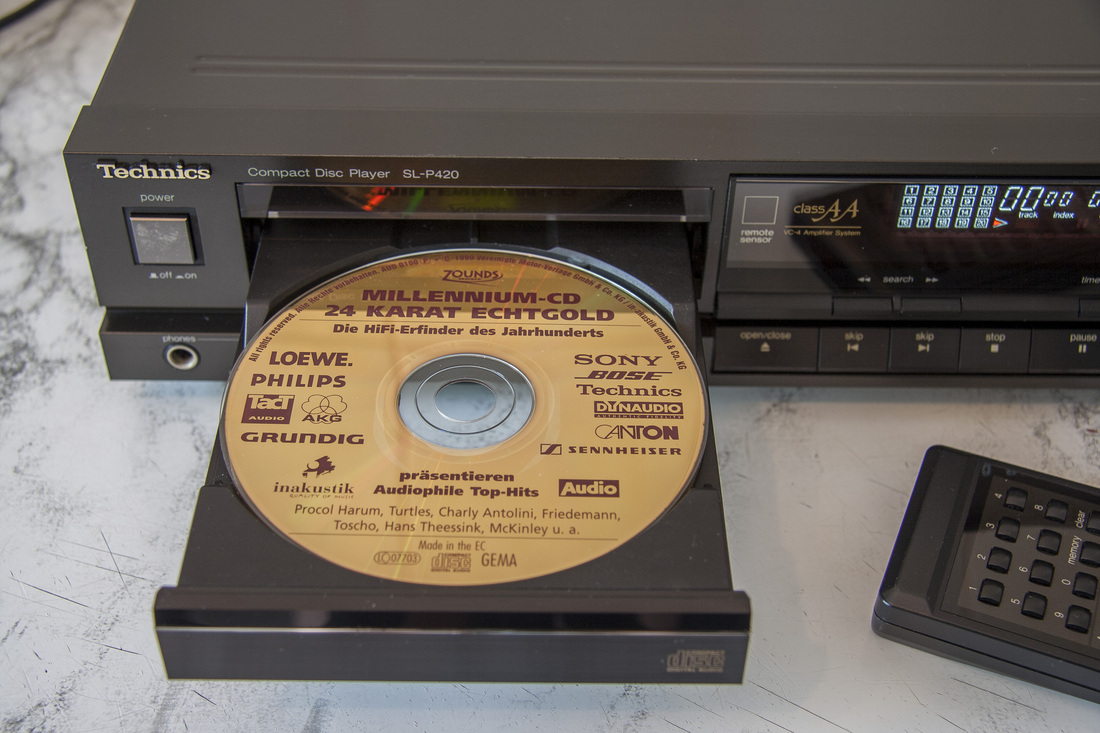The image depicts an indoor setting with a white marble countertop featuring black streaks and some scratches. Centered on the countertop is a vintage, grayish-black, front-loading Technics Compact Disc player, model SL-P420, likely from the late 80s or early 90s. The CD tray is open, revealing a gold-colored CD labeled "Millennium CD 24 Karat Gold," adorned with numerous logos and text, including brands like Sony, Bose, Technics, and more, along with some German words.

In the upper left corner of the CD player, "Technics" is written in gold font, with a white "Compact Disc SL-P420" label above the disc door. Below the Technics logo, the word "Power" is printed in white, accompanied by an on/off switch. The front panel features a variety of buttons for functions such as open/close, skip, stop, and pause. On the right side, there is a digital display panel with greenish lighting, indicating track information.

Additionally, a small, vintage remote control with numbered buttons is situated near the player. The neat arrangement and well-maintained appearance suggest the player is in good condition, despite its age.